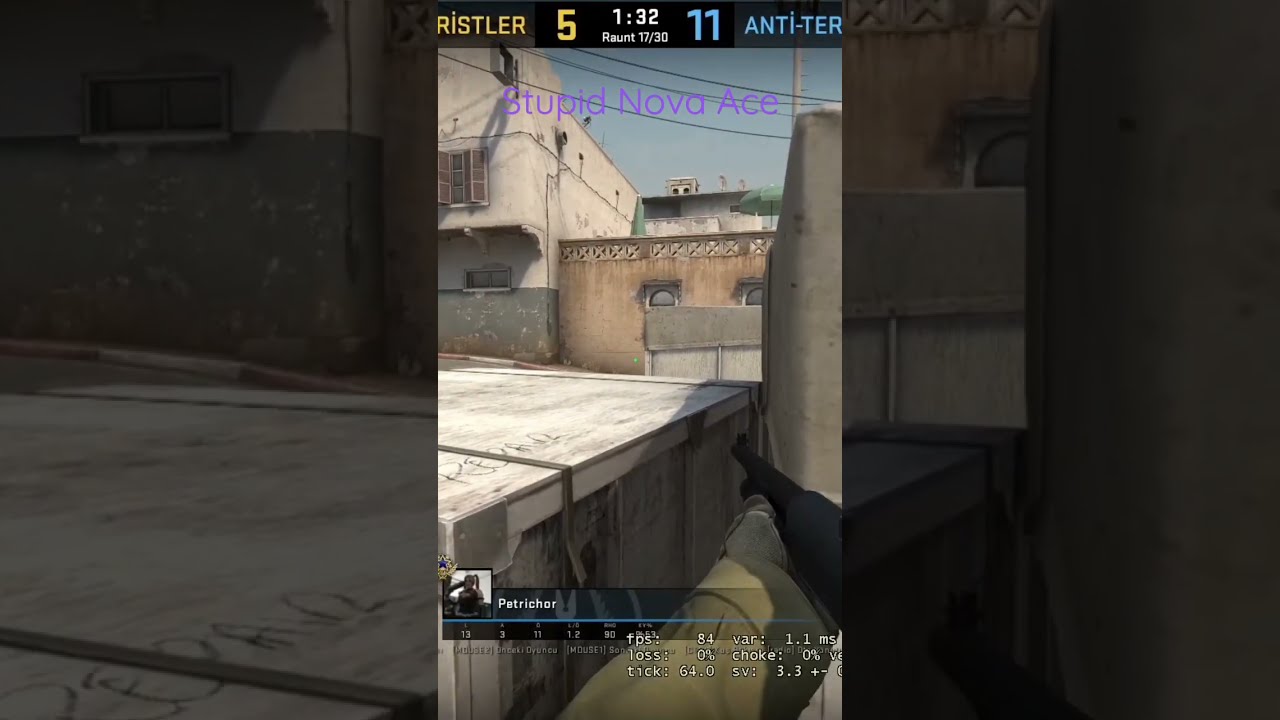This detailed composite description centers around a vertical screenshot of a first-person shooter mobile video game, flanked by darker, zoomed-in close-ups on both sides. The scene, set on a rooftop in the Middle East, captures the player's perspective, aiming a black rifle towards various stone buildings. The soldier, depicted in an olive green uniform with matching gloves, points the gun towards a tan building, while a gray building is visible to the left. At the top of the display, game details include "Ristler 5-132" and "round 17 out of 30," with "11 anti-tier" representing the opposing team. The clear, blue sky peaks in the top right corner. Prominently displayed in purple text is the username "stupid.nova.ace." Below the main action, a scoreboard featuring the soldier’s logo and stats is visible. All elements of the game are presented upright within the confines of a cropped portrait view, with the overall composition revealing an immersive urban combat environment.